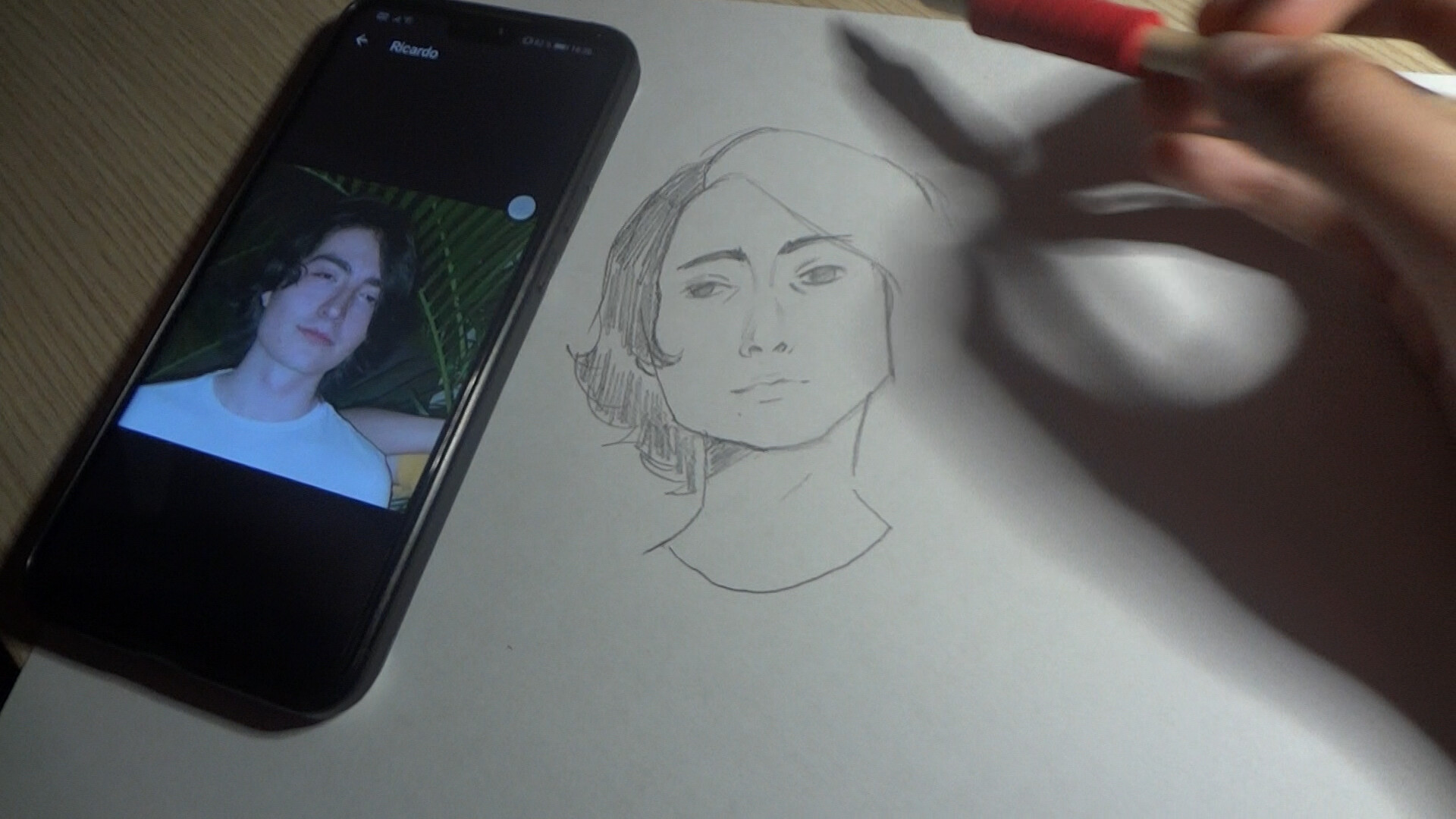In the upper right corner of the image, a Caucasian hand is seen delicately gripping a pencil, actively sketching on a piece of pristine white drawing paper. Positioned beside the hand is a cell phone displaying a photo of a young man with dark hair and wearing a white t-shirt, who appears to have a somewhat foreign look. The hand appears to be skillfully replicating the young man's selfie onto the paper, with the initial outlines and details of the sketch already taking shape, showcasing an intimate moment of artistic creation.